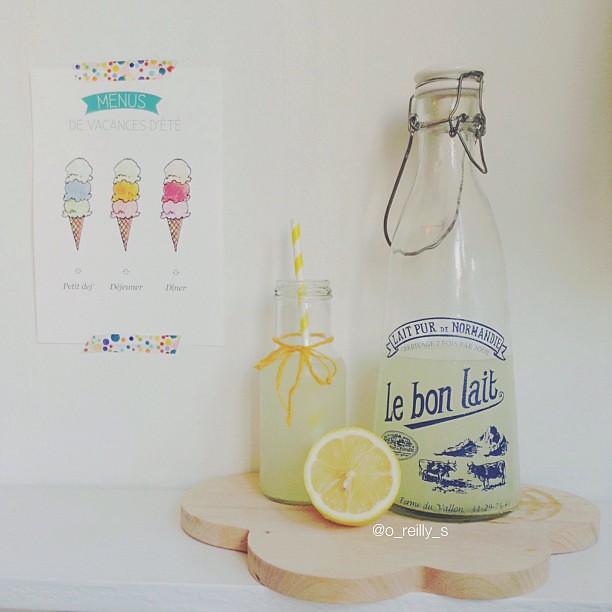The image features a clear, old-fashioned glass bottle with a metal clip and a white top, labeled "Le Bon Lait" in blue, adorned with blue illustrations of cows and other designs. The bottle is about halfway filled with lemonade and stands on a flower-shaped wooden cutting board. Positioned to the left of the bottle is a halved lemon, oriented towards the camera. Adjacent to the lemon is a shorter, drinking bottle, also partially filled with lemonade, decorated with a yellow and white striped straw and wrapped with yellow twine. The entire setup sits against a white background. Hanging on the wall in the background is a menu titled "Menus de Vacances d'Été," featuring three images of ice cream cones, each with three scoops of different colored ice cream. The menu is affixed to the wall with white tape, which has multicolored polka dots.